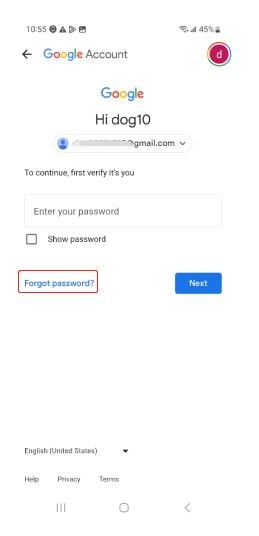The image displays a digital interface at a time of 10:55, with a few icons visible on the right side, one indicating a 45% battery level. On the left of the screen, there is a back arrow pointing to the left, followed by the text "Google account" adjacent to a purple circle with the letter "C" in the middle. Below this, the Google logo is present, featuring the multicolored letters G (blue), O (red), O (yellow), and G (green). Underneath, there's a salutation saying "Hi dog 10," followed by an email address partially blurred out for privacy, continuing with "@gmail.com." Further down, the screen prompts the user to "continue first, verify issue," accompanied by a text field labeled "Enter your password." Adjacent to this, an unchecked checkbox is labeled "Show password." Below this, a blue hyperlink reads "Forgot password." Additionally, the email and password fields are outlined with a red rectangular box. Lastly, on the right side of the screen, there's a dark blue button labeled "Next."